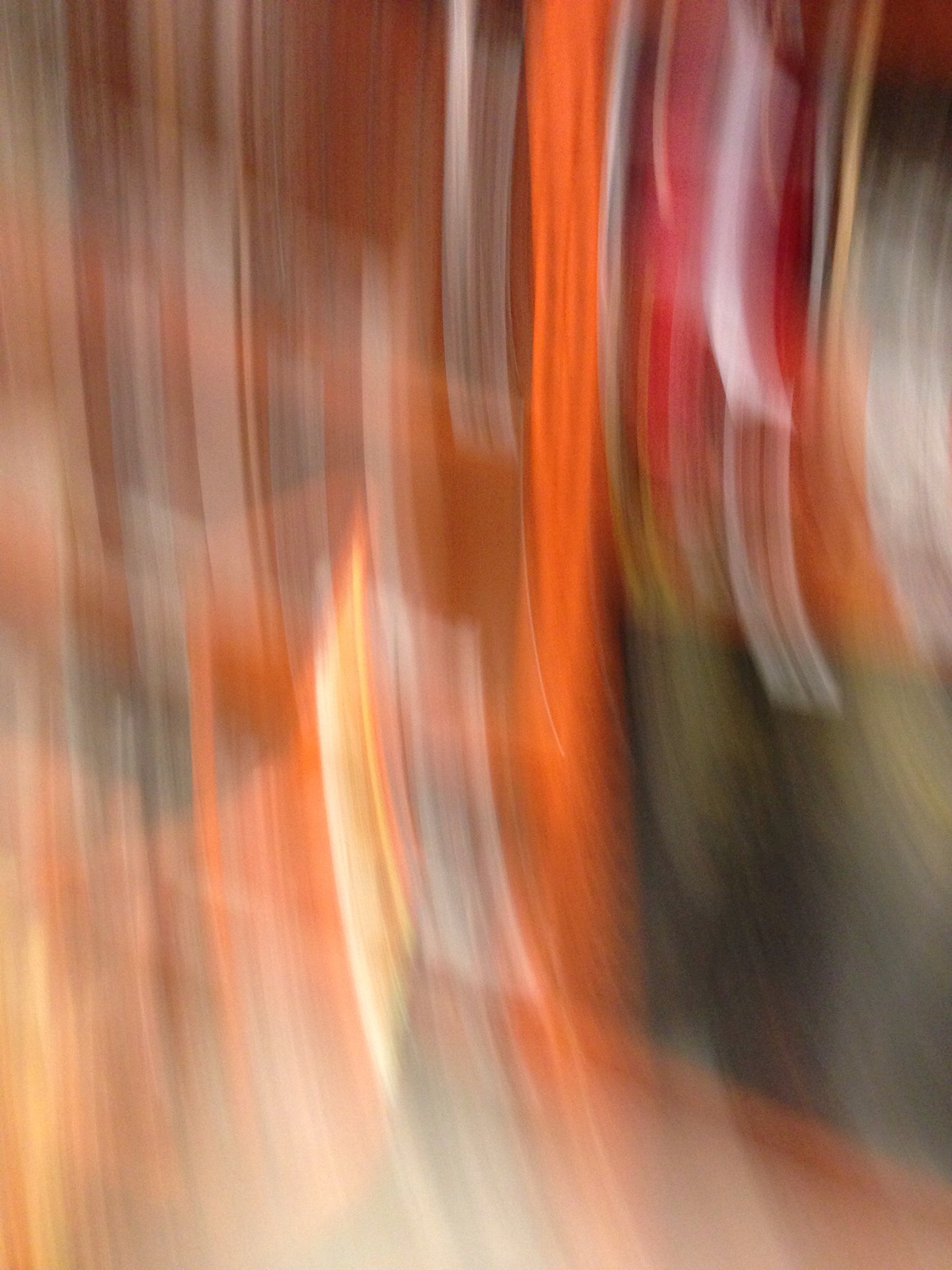This photograph is an abstract, heavily blurred image characterized by dynamic streaks of light and color. The composition features predominantly shades of red, orange, and white, with additional hints of black and brown. The colors streak vertically, swirling slightly to the right in certain sections, mimicking the effect of a long-exposure shot taken from a moving car capturing city lights. The right of the center is dominated by a prominent bright orange streak that extends from the top and fades towards the bottom. Just left of this, a darker orange streak transitions into a brighter orange midway down the image. Below this area, bright white and yellow streaks can be seen. To the right, a red streak appears midway, morphing into green before disappearing. The overall effect resembles an impressionistic watercolor painting with random yet aesthetically pleasing arrangements of colors and textures. No discernible objects or text are visible, leaving the image as a pure study of light and movement.